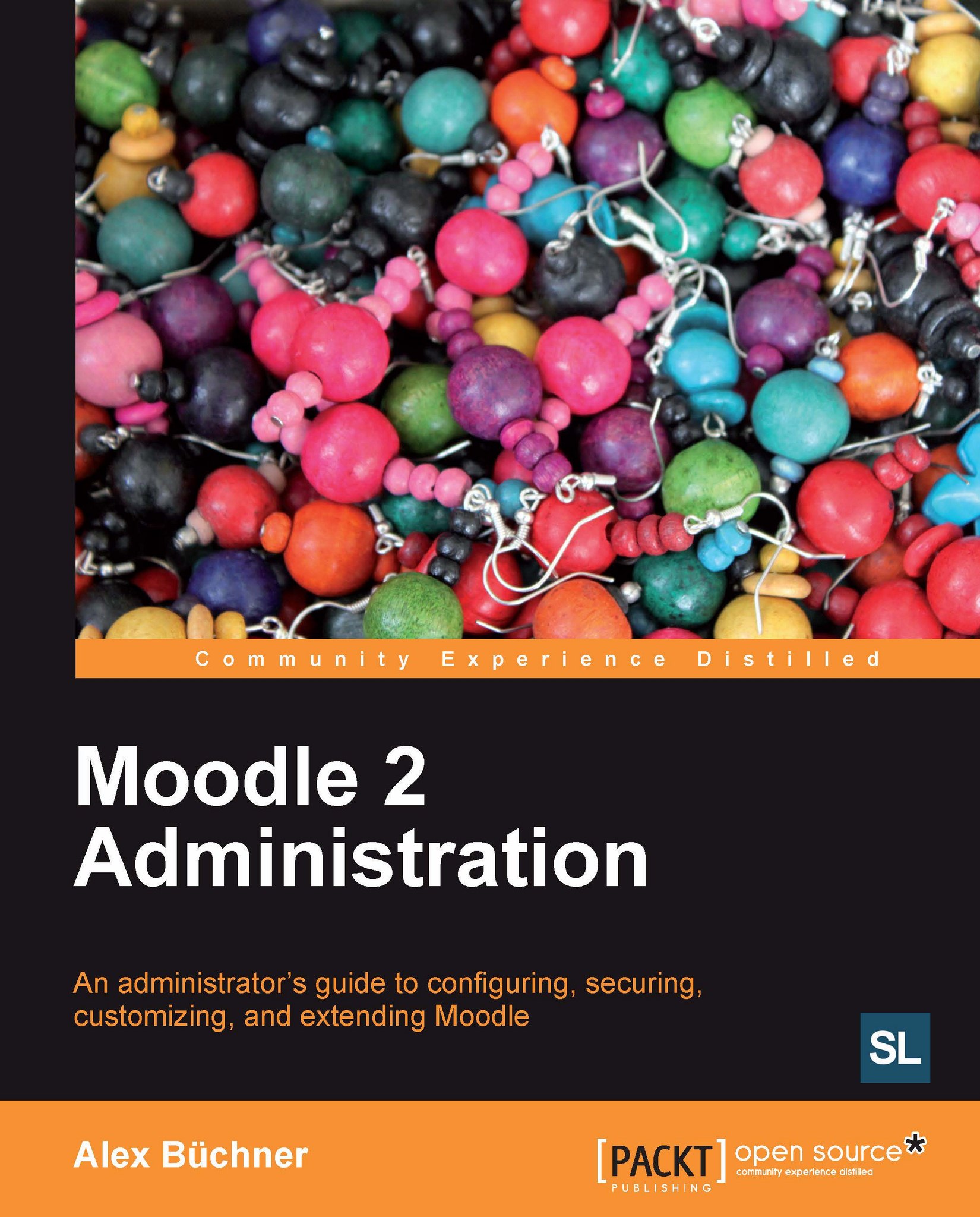The image depicts the front cover of a book titled "Moodle 2 Administration: An Administrator's Guide to Configuring, Securing, Customizing, and Extending Moodle" by Alex Buchner, published by Packt Publishing. The cover features a vibrant photograph of handmade, multicolored beaded earrings in shades of pink, black, orange, red, green, yellow, and more, arranged in a pile towards the top. An orange banner at the bottom lists the author's name and the publisher, Packt Publishing Open Source, with the text "Community Experience Distilled" prominently displayed. The background of the cover is black, accentuating the colorful beads and the orange text bars.